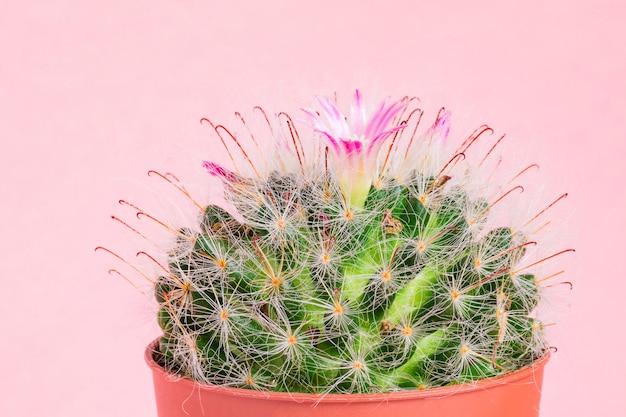The image portrays a vibrant, green, dome-shaped cactus, prominently positioned in a pink or orange pot against a light pink background. The cactus is adorned with numerous yellow and white spikes, interspersed with fine, hair-like orange filaments. Emanating from the center of the dome is a striking purple flower, which has a yellow base and tulip-like petals that are purple with stripes. Additionally, there are smaller reddish protrusions emerging from the cactus, adding intricate detail to its appearance. The overall composition closely resembles a painting, with the detailed textures and vivid colors creating a captivating, close-up view of the flowering cactus.